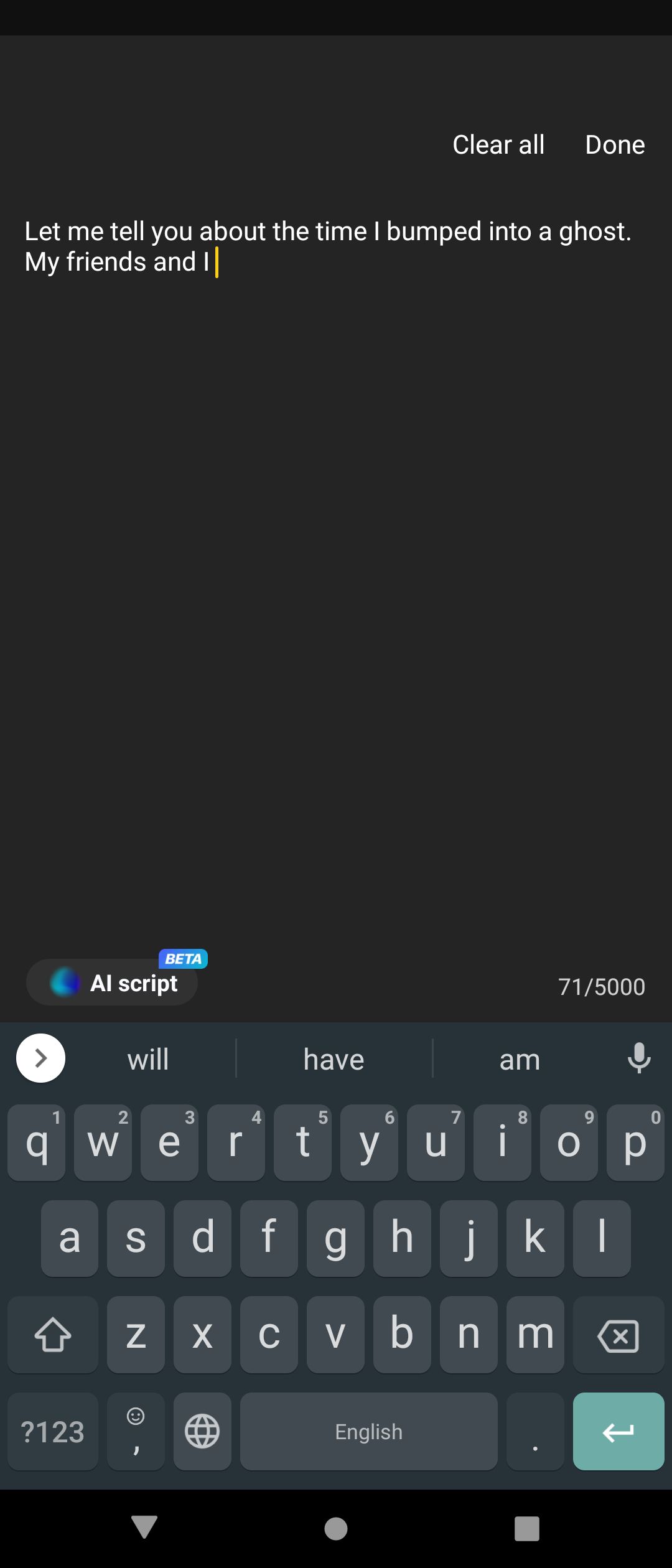In this image, the top section displays a partially typed message that reads, "let me tell you about the time I bumped into a ghost, my friend and I," with a yellow line appearing after the word "I," indicating an unfinished typing process. The text is white and set against a black background. Positioned to the right above this line of text are the options "clear all" and "done."

At the very bottom of the image, there is a visible keyboard featuring all the letters of the alphabet. Additional keys include a backspace (or erase) button, a back arrow, a microphone icon for voice input, an up arrow, and a "1, 2, 3" button for numerical input. There is also a smiley face icon, presumably for accessing emojis.

Further down at the lowest part of the image, three distinct shapes are visible: an upside-down triangle on the left, a circle in the middle, and a square on the right. These symbols suggest that the image is a screenshot taken from a smartphone, likely an Android device.